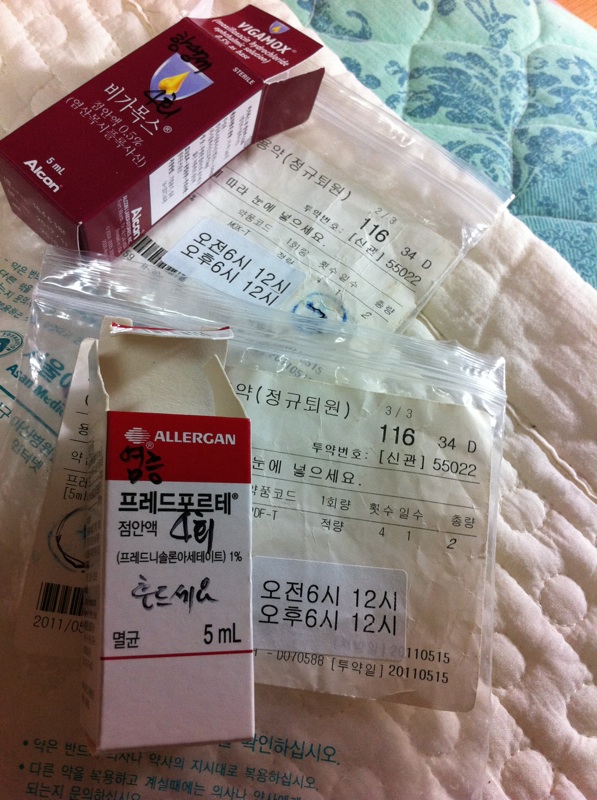This close-up photograph depicts two medicine boxes and some additional items arranged on a quilted white bedspread, which lies over a blue and green floral-patterned mattress. The box on the left is maroon with white writing that reads "Vigamox" and features an image of a golden teardrop inside a bowl, flanked by Japanese text, and marked with "5ml" at the bottom alongside the brand name "Alcon" in white. The white and red box, labeled "Allergan" at the top in a red square, also displays Japanese text and "5ml" in black. Both boxes are open and placed on their sides, resembling small milk cartons. Behind these boxes are two Ziploc bags containing yellowed papers, perhaps bills of lading or instructional sheets. The detailed scene captures the items against the backdrop of a white bedspread, partially pulled back, with the edge of a wood floor visible on the right.